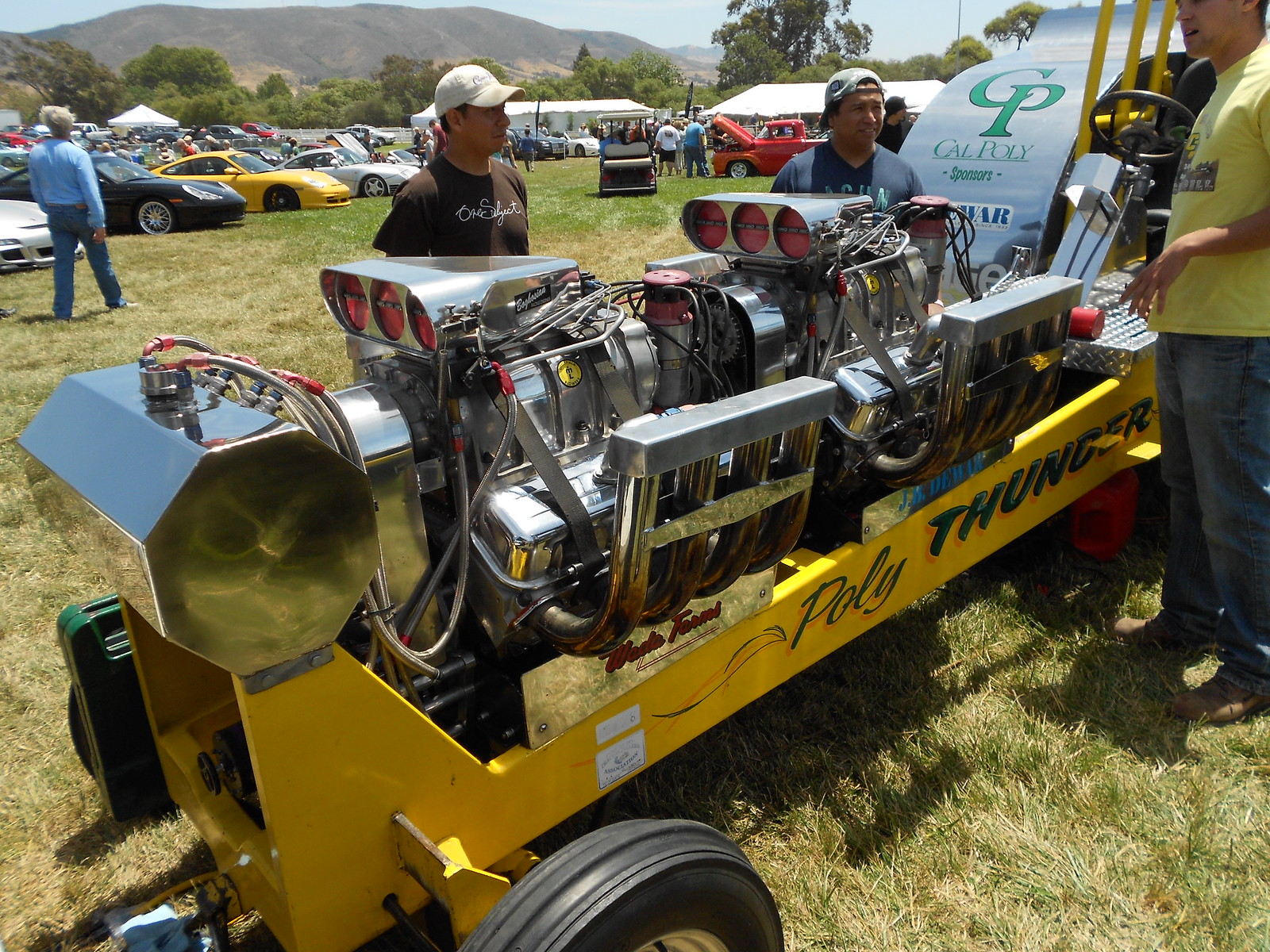The digital photo captures an outdoor scene at what appears to be a lively car show held on a sunny day, in a vast open field with a scenic mountainous backdrop and lush green tree line. Front and center is a distinctive homemade hot rod, mounted on a yellow wagon-like structure with wheels. The hot rod, featuring two silver engines stacked, prominently displays the name "POLY THUNDER" on its side in cursive black and capital letters. Beside the hot rod, a sign reads "CP Cal Poly Sponsors" in white font on a green and black background. Surrounding this focal point are a variety of parked sports cars - notably, a yellow one, a black one, and two white ones. Several men are seen in casual attire, engaging in conversation near the hot rod and sports cars. Among them, a man in a yellow shirt paired with blue jeans, and men in white caps - one is worn backwards and another forwards. Additionally, a man with salt and pepper hair wearing a blue long-sleeved shirt and jeans walks away from the scene. The atmosphere is bustling, capturing the essence of a vibrant community event.